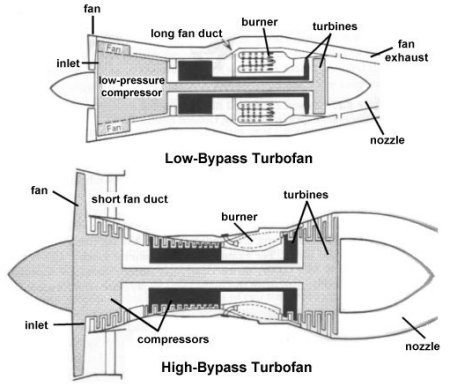This detailed black and white infographic illustrates two stages of turbofan engines, depicted from both bird's-eye and side views. The top portion shows a labeled diagram of a low bypass turbofan, highlighting components such as the fan, long fan duct burner, turbines, fan exhaust nozzle, low-pressure compressor, and inlet. In contrast, the bottom portion features a detailed depiction of a high bypass turbofan, also meticulously labeled with its key parts including the fan, short fan duct, burner, turbines, nozzles, compressors, and inlet. Both diagrams are rendered in shades of gray and dark black on a white background, arranged horizontally in a square format with labels in black text. The image is technical and educational, resembling a pamphlet designed to elucidate the key differences and components of turbofan engines.